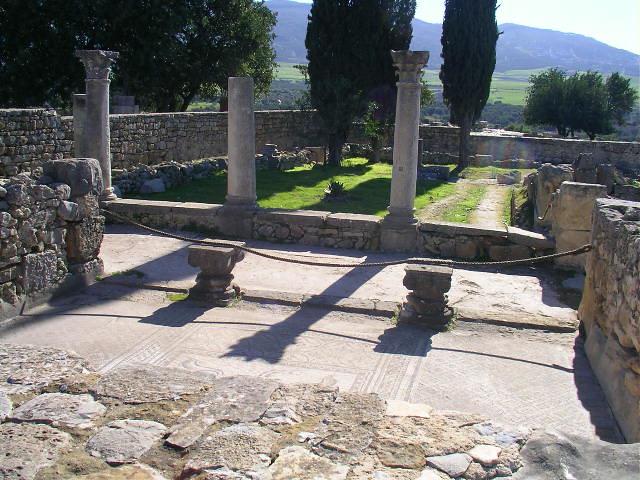In this detailed image taken outdoors, likely during the middle of the day, we see a historic setting featuring ancient stone structures that seem to date back to Roman times, possibly with elements of Greek architecture. The setting includes a stone staircase leading down to a centrally positioned stone walkway. The walls and columns are made of gray stone, indicative of ancient construction. A rope, or possibly a chain, blocks entry to a specific area between the bases of columns, acting as a barrier to keep people out.

Surrounding this central stone area is a grassy field with clusters of tall trees towards the center and center-left of the image, and large, forested hills in the distance. The sky appears slightly hazy, but the sun is out, casting sharp, long shadows across the scene. The various colors present in the image include different shades of tan, brown, gray, white, and green, enhancing the rustic and historic ambiance. The image conveys a sense of an ancient, possibly Roman, outdoor space, marked by classic architectural elements and a serene, natural setting.